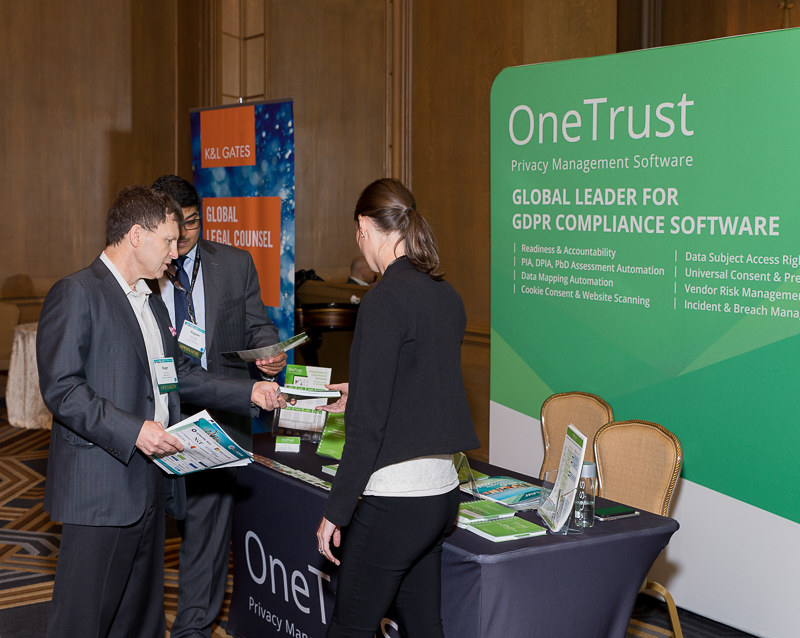In a bustling interior space of a large venue, a tech trade event unfolds, drawing professionals from various sectors. At the heart of the photograph, three individuals are deeply engaged in conversation, epitomizing the spirit of networking and business exchange. The two gentlemen on the left, one with a white complexion and the other of Indian descent, both dressed in black suits with short hair, converse earnestly with a woman standing between them, her hair tied back and also clad in a black suit. The trio, all holding pamphlets, stands in front of a table adorned with a black cloth bearing the branding of OneTrust, a leading company in privacy management software. Behind them, a vibrant green banner with white text proudly announces "Global Leader for GDPR Compliance Software," detailing various specialties like readiness and accountability, PIA, DPIA, PBD, assessment automation, data mapping automation, cookie consent, and web scanning. Additional advertisements, including one for KBL Gates with orange and blue elements, add to the dynamic atmosphere, emphasizing the diverse array of companies participating in this event.